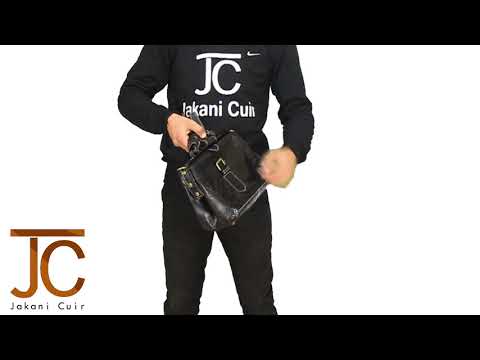The image centers on a standing male figure, predominantly dressed in a black outfit consisting of a long-sleeved shirt and black pants. His shirt features the Nike logo beside the initials "JC," and below that, the words "Chikani Cure" appear in white font, giving it a unique fashion design flair. He is holding a sleek black leather bag with straps in his right hand, while his left hand is engaged in opening a portion of the bag, possibly a side zipper. Notably, the image contains the JC initials with "Chikani Cure" beneath them in brown and orange font in the lower left corner, suggesting a branding element. The background is white, framed with horizontal black lines at the top and bottom, adding to the minimalist, stylish presentation of this personal advertisement, likely for a modeling agency or a fashion business.